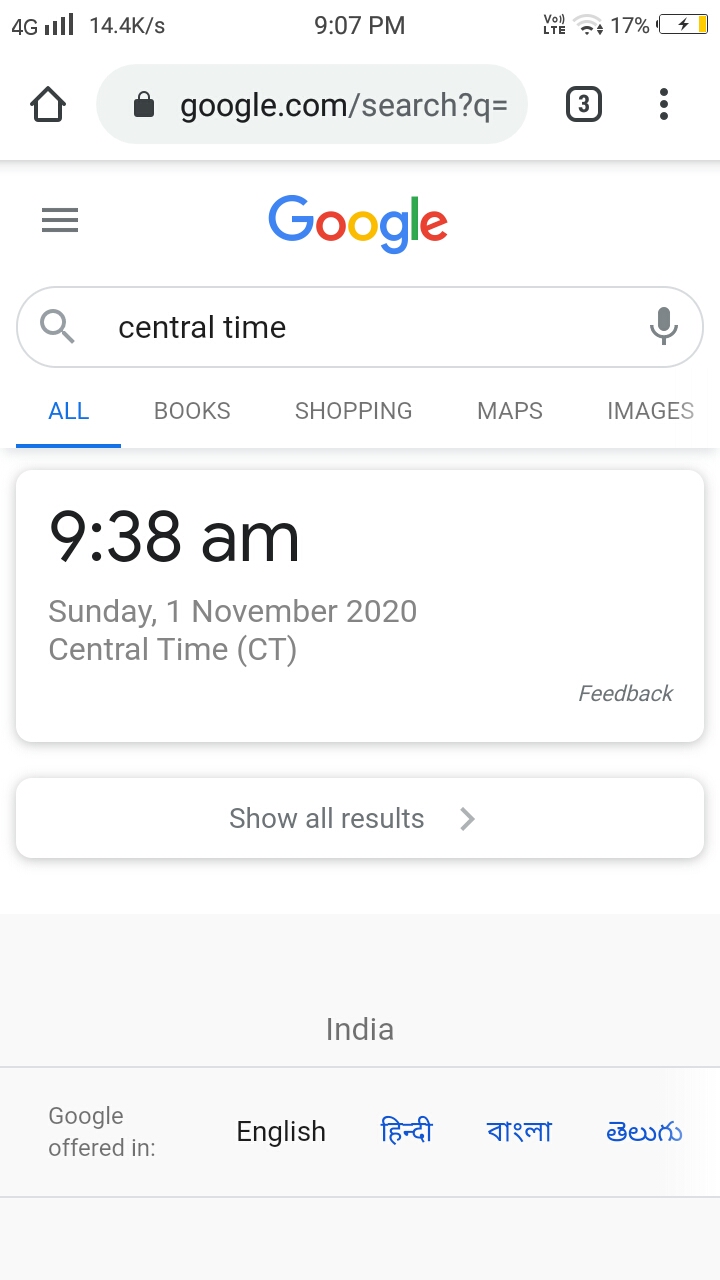The image depicts a smartphone screen displaying the Google search page. In the top-left corner, the status bar shows that the device has a 4G connection with full service bars. To the immediate right, it displays the time "9:07 PM" in the middle of the status bar, followed by the Wi-Fi icon and the battery icon indicating the phone is at 17% charge and is currently charging, with the percentage highlighted in yellow.

The browser address bar at the top reads "google.com/search." Below this, there's an interface showing a home icon, a square containing the number three, and a three-dot menu icon. The prominent Google logo on the page is presented in its traditional colors: blue, red, yellow, blue, green, and red.

Within the search bar, the query "central time" is entered, accompanied by a microphone icon on its right. The search results indicate that the current time is "9:38 AM" on "Sunday, November 1st, 2020," listed as "Central Time (CT)." Immediately beneath this, there's a prompt displaying "Show all results" with a right-pointing arrow, followed by the words "India" and "Google offered in: English."